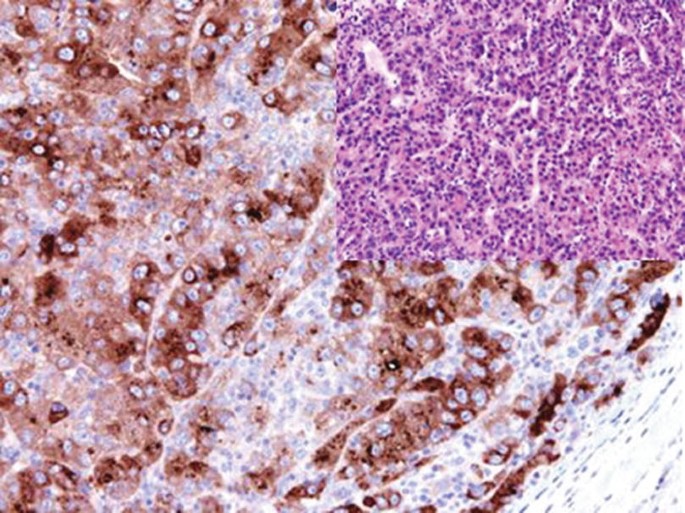This color photograph appears to be an extreme microscopic close-up of a sample, possibly biological in nature. Dominated by swirls and splotches, the main part of the image features a marbled texture with rust-colored reds, light bluish, purplish-gray hues, and extensive brown and white areas. The photograph is rectangular, and within the top right corner, there is a distinct square inset characterized by a mix of pink, white, and purple tones. This area contains numerous purple dots and white streaks, evoking the appearance of cellular or bacterial structures. Vein-like patterns are also present, adding to the intricate and wild marble-like appearance. Although reminiscent of a science book illustration or a countertop, the exact nature of the sample remains unidentified due to the lack of any textual explanation.